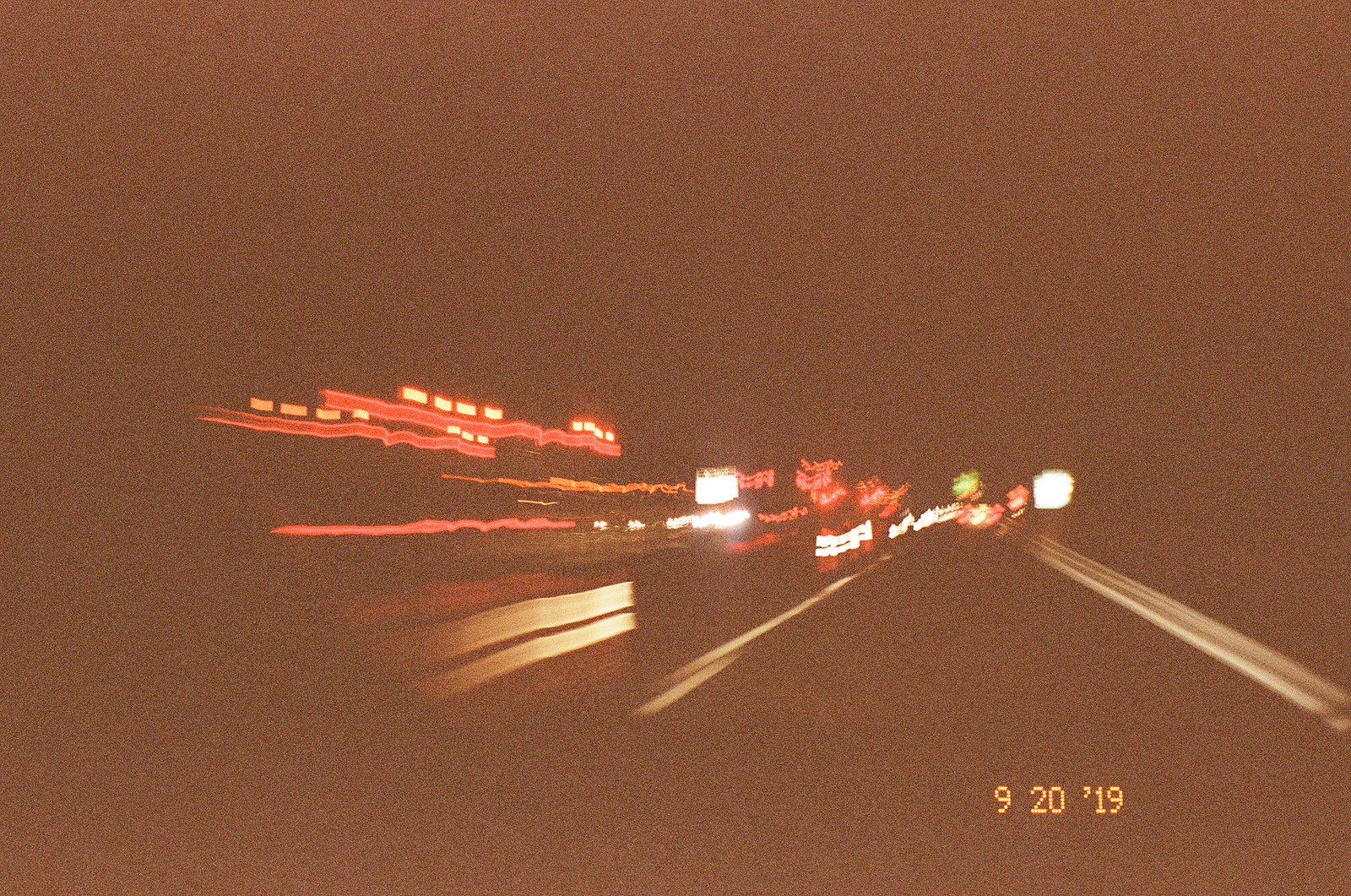The image depicts a nighttime urban scene characterized by a mid-brown rectangle area. In the foreground, a well-lit road enters from the right and intersects with another roadway. Prominent buildings on either side of the intersection glow with bright white lights illuminating their facades. Behind these structures, additional buildings are visible, casting a pink hue for reasons not clear in the image, possibly due to filters. Leading into the backdrop, a wide road described as a "brown double streak" stretches off towards the left, indicating the directionality and flow of urban traffic. While several buildings feature the same white lights, the dominant pink coloration adds an unusual, almost surreal, visual element to the scene.